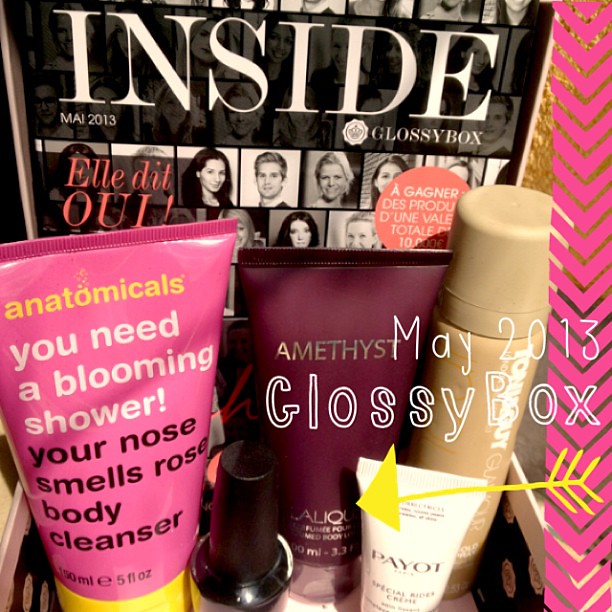The image depicts a curated subscription box, specifically the May 2013 Glossybox, which features various cosmetic products. The lid of the box includes the text "May 2013 Glossybox" in a girly font, alongside headshots of several individuals, potentially celebrities. The products inside are meticulously arranged, with a notable use of digital overlays, including pink and yellow arrows pointing to specific items. The most prominent product highlighted by a yellow arrow is a burgundy squeezable tube labeled "Amethyst." On the left side of the box is a pink tube labeled "Anatomicals: You Need A Blooming Shower - Your Nose Smells Rose Body Cleanser," presumably a 5-ounce body cleanser. Additional items include a small white tube, a light brown cylindrical canister, and a nail polish or nail polish remover. Overall, the presentation is vibrant and meticulously curated, with an emphasis on the detailed labeling and digital annotations enhancing the visual appeal of the featured products.